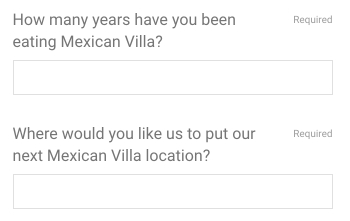In the image, there is a white background featuring text fields that pose a couple of questions to the viewer. The first question asks, "How many years have you been eating Mexican food?" The second question inquires, "Where would you like us to put our next Mexican villa location?" The latter is labeled as a required field, but it is currently empty. The setting is clean and minimalist, with the repetitive emphasis on the latter question highlighting its importance in the survey.